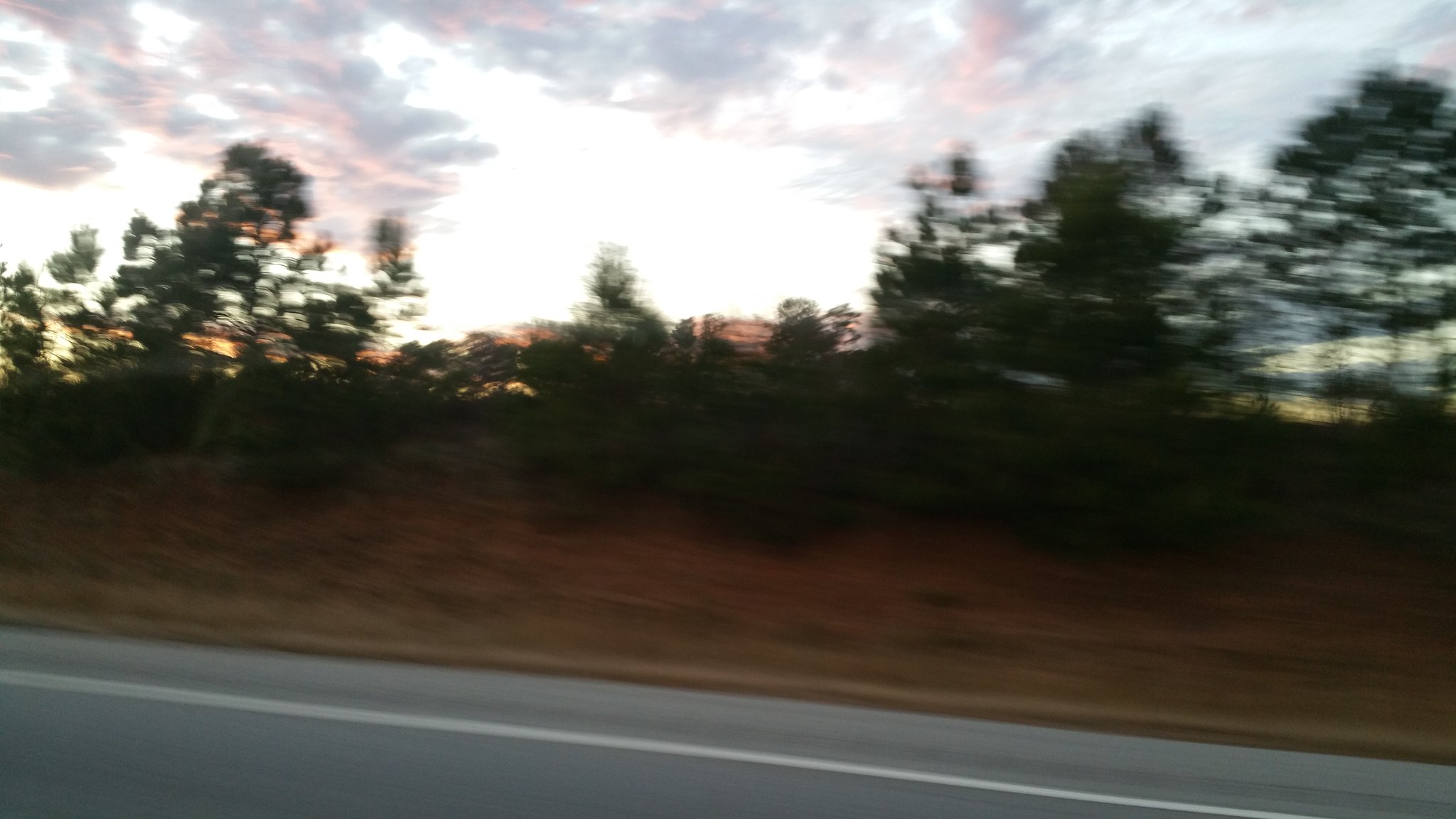This photograph, taken from a moving vehicle, captures a slightly blurry scene of a roadside at sunset. The road, visible at the bottom of the rectangular frame, features a dark gray pavement with a distinct white stripe dividing the driving lane from the shoulder. The roadside is characterized by a brown embankment, suggesting either winter grass or bare earth. Rising from the top of the embankment, a row of various green trees, possibly including conifers, stretches across the image. The background showcases a dramatic sunset sky, with a faint light blue that darkens towards the right. The sky is adorned with ominously colored clouds—gray, blue, and off-pink—with some appearing reddish on the undersides, indicating the setting sun towards the far left. This roadside scene captures the essence of motion and the transitional beauty of twilight as seen from the window of a moving car.